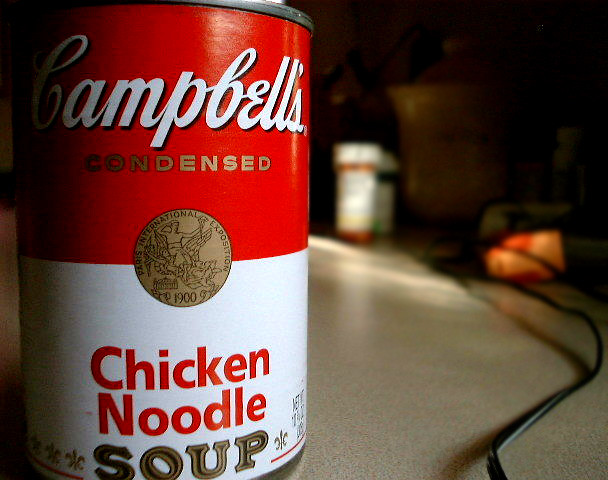This image features a can of Campbell's Condensed Chicken Noodle Soup prominently displayed. The can's classic white and red label showcases the Campbell's logo and an iconic emblem centered within the design. In the middle of the label, there's a detailed illustration, possibly depicting a character lounging with one arm behind their head while the other is raised. Surrounding this emblem, elegant text reads "International Exposition," adding a historic touch.

The can is placed on what appears to be a kitchen counter or table. To the side of the can, a thin wire extends vertically out of the frame, while in the background, two medicine bottles can be seen blurred out, indicating they are not the focal point. The clean and organized setup serves to highlight the classic design and nostalgic feel of the Campbell's soup can.